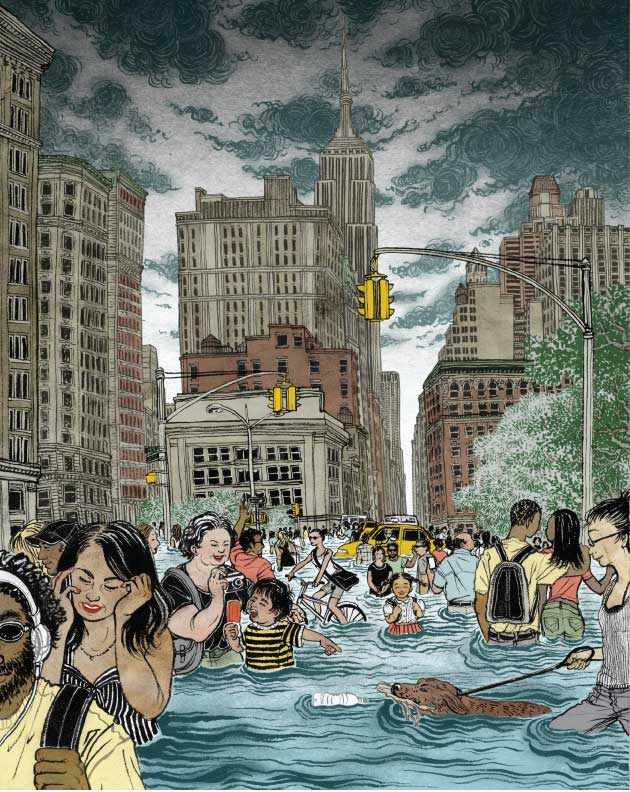This vertically aligned rectangular drawing portrays a chaotic urban flood scenario. The top of the image features a tumultuous sky filled with swirling gray and white clouds, casting an ominous tone over the scene. Below the unsettled sky, the cityscape is dominated by tall brown stone buildings that stretch across the middle section of the image. Streetlights and traffic poles are sporadically placed, with one spotlight hanging over the center from the right and a traffic light positioned similarly on the left.

Amidst the floodwaters, which reach up to an adult's waist and a child's stomach, the city’s inhabitants react in various ways to their submerged surroundings. Some pedestrians appear distressed, such as a woman in the left corner who cups her face in despair. In contrast, others seem oddly unfazed by the calamity: a child eating a popsicle, his mother capturing the moment with her camera, and several people walking leisurely or bicycling through the flood, some even smiling. In the background, a yellow taxi maneuvers through the water, while on the right, trees stand conspicuously unaffected by the flood.

Details like a swimming dog, floating debris, and a bottle add to the sense of a city grappling with an unexpected deluge. Despite the clear evidence of disaster, the mixture of nonchalant and distressed reactions creates a surreal, almost dystopian atmosphere.